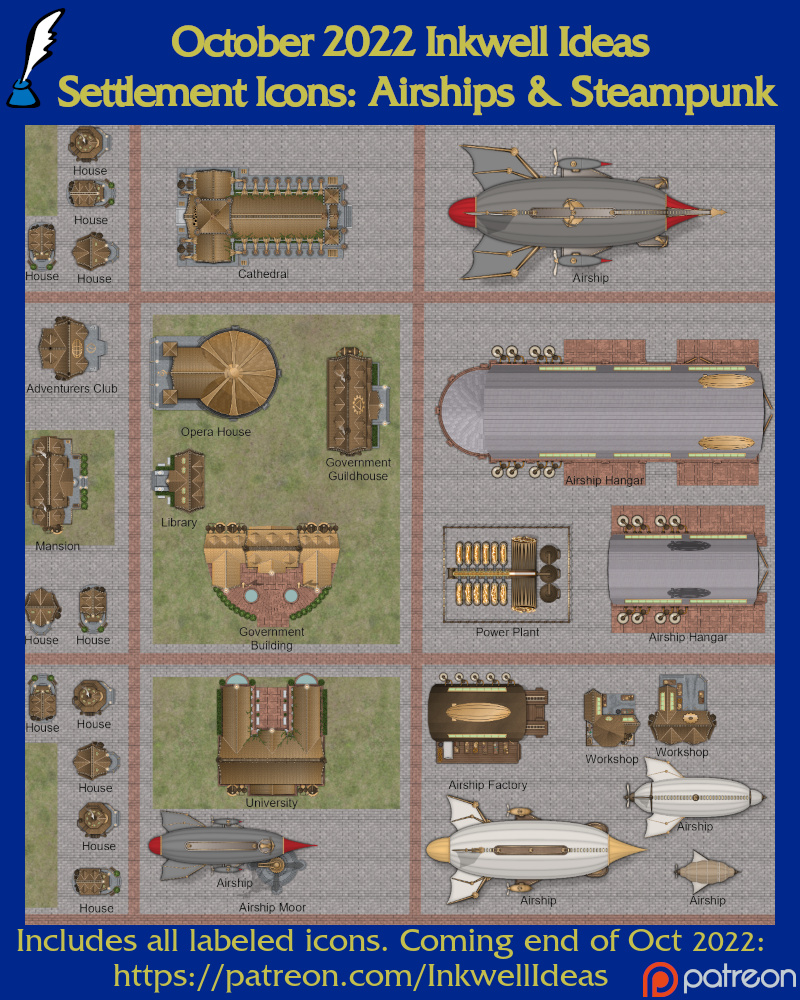The image is a detailed poster featuring a blue border that is thicker at the top and bottom and thinner on the sides. In the upper left corner, there is an icon of a blue inkwell with a white feather. The top of the poster reads "October 2022 Inkwell Ideas" in yellow font, followed by "Settlement Icons: Airships and Steampunk." Below this heading, the poster is divided into three columns, each containing three rectangles with various labeled illustrations of airships and steampunk elements. These images are spread across the columns with accompanying text too small to read. At the bottom of the poster, also in yellow font, it states, "Includes all labeled icons, coming end of October 2022." Below this is the URL "https://patreon.com/inkwellideas" with a Patreon logo and the word Patreon in white located in the bottom right corner.